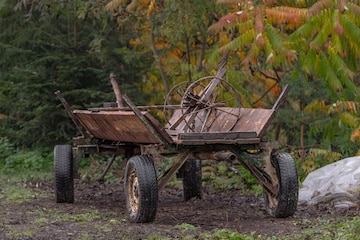This small, cropped, horizontal photo depicts a historic, wooden cart situated on a dirt pathway within a wooded area. Unlike a traditional wheelbarrow, this cart features four large wheels, one at each corner, rather than three, and lacks a handle. The cart has a flat bed with sides projecting outwards slightly, giving it a catty-cornered appearance. Made from natural wood, it rests on the ground appearing somewhat dirty with caked-on dirt. Atop the cart, there are two large, old wheels that resemble oversized bicycle wheels or wagon wheels, but without rubber tires, possibly serving as spare wheels. To the right of the front left wheel, a large boulder is visible. The surrounding scenery includes lush greenery and shrubs, with some trees showing hints of fall colors, suggesting the image was captured during autumn.